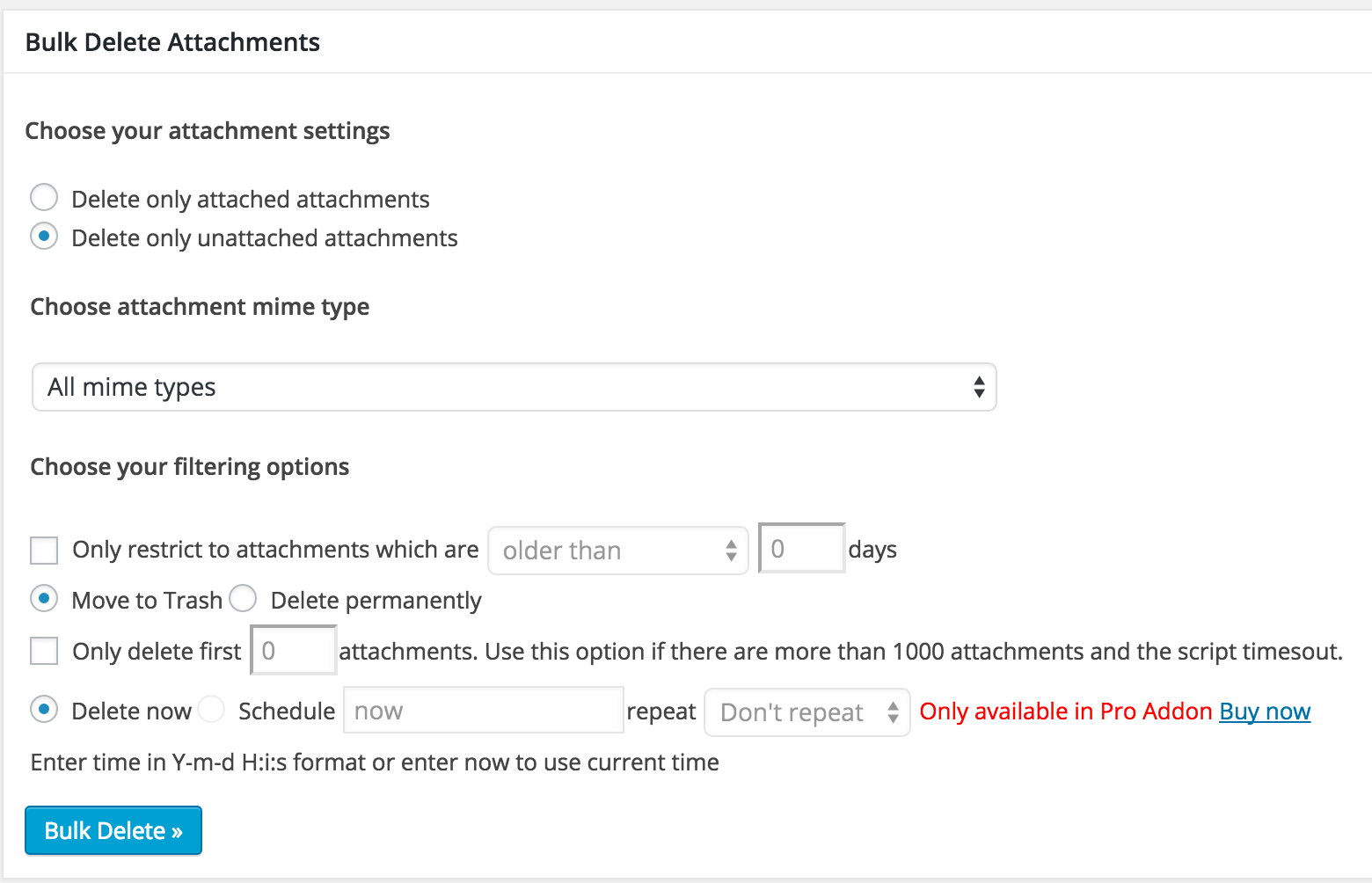A detailed screenshot displays a pop-up interface titled "Bulk Delete Attachments." This interface is designed to facilitate the mass deletion of attachments and contains multiple configuration options for the user to specify their preferences.

At the top, the title "Bulk Delete Attachments" is prominently displayed in bold text, signaling the purpose of the window. Directly beneath the title, several subheadings with associated options are provided to refine the deletion criteria.

The first subheading, "Choose your attachment settings," offers two radio button options: "Delete only attached documents" and "Delete only unattached documents," with the latter option currently selected and highlighted by a blue dot.

The next subheading, "Choose attachment MIME type," presents a drop-down menu with various MIME types to choose from. The default selection, "All MIME types," is currently active.

Below this, another subheading, "Choose your filtering options," lists several criteria, some of which are optional and some pre-filled. Options include "Move to trash," which has been selected, "Delete now," which is checked, and one unfilled criterion. Another unselected option indicates it is only available in the "Pro add-on" with accompanying red text emphasizing this limitation.

At the bottom of the interface, users are prompted to "Enter time" in the format YYYY-MM-DD HH:MM:SS, with an option to use the current time by leaving these fields blank.

The window is styled in a minimalist fashion with a white background and black text, accented by blue elements indicating selection. A notable blue button labeled "Bulk Delete" sits at the bottom, ready to execute the configured actions. Hyperlinks within the interface also appear in blue, maintaining consistency.

Overall, this straightforward interface clearly outlines the steps and options available for bulk deleting attachments, making the process user-friendly and efficient.